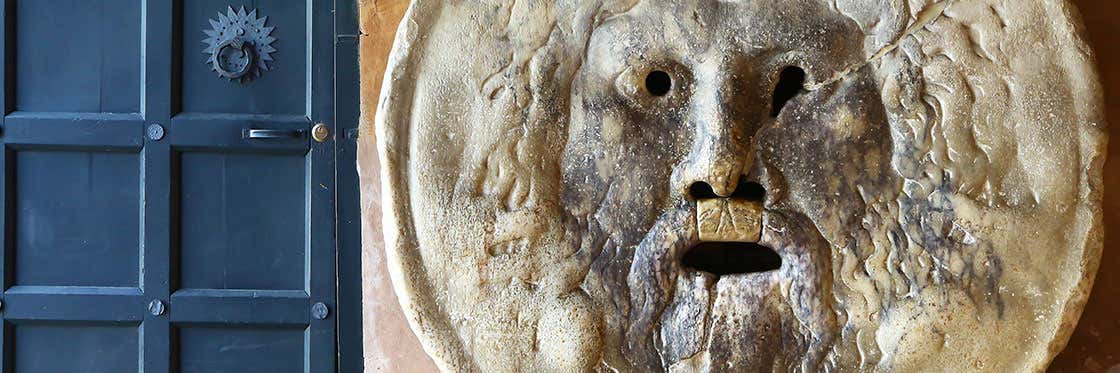The image shows a large, circular piece of art resembling a face, mounted on a wall. The piece has the appearance of a ceramic plate with a raised edge, predominantly light cream in color around the border. Its top and bottom are partially obscured by the wall's edges. The central section is marked by blue and purple lines, giving it a somewhat ghastly appearance. Two asymmetrical eye holes contribute to this effect: the left eye is surrounded by an orange tint and shaped like a round hole, while the right eye is an upside-down teardrop shape in black. A crack extends from the right eye towards the upper left corner of the piece. Below the eyes, the nose features two black holes with a copper hue at the tip. The mouth is represented by an oval-shaped, black hole.

Adjacent to the artwork, on the left, is a blue door with a grid pattern of panels. It features a blue door handle, a golden button, and a sun-shaped knocker with a solid blue ring in the center. The wall itself has an adobe-like texture, painted in an orange color, enhancing the earthy look. The entire scene, combined with the distorted face and the aged, icy appearance, invokes a sense of an ancient, ghostly presence embedded within the wall.